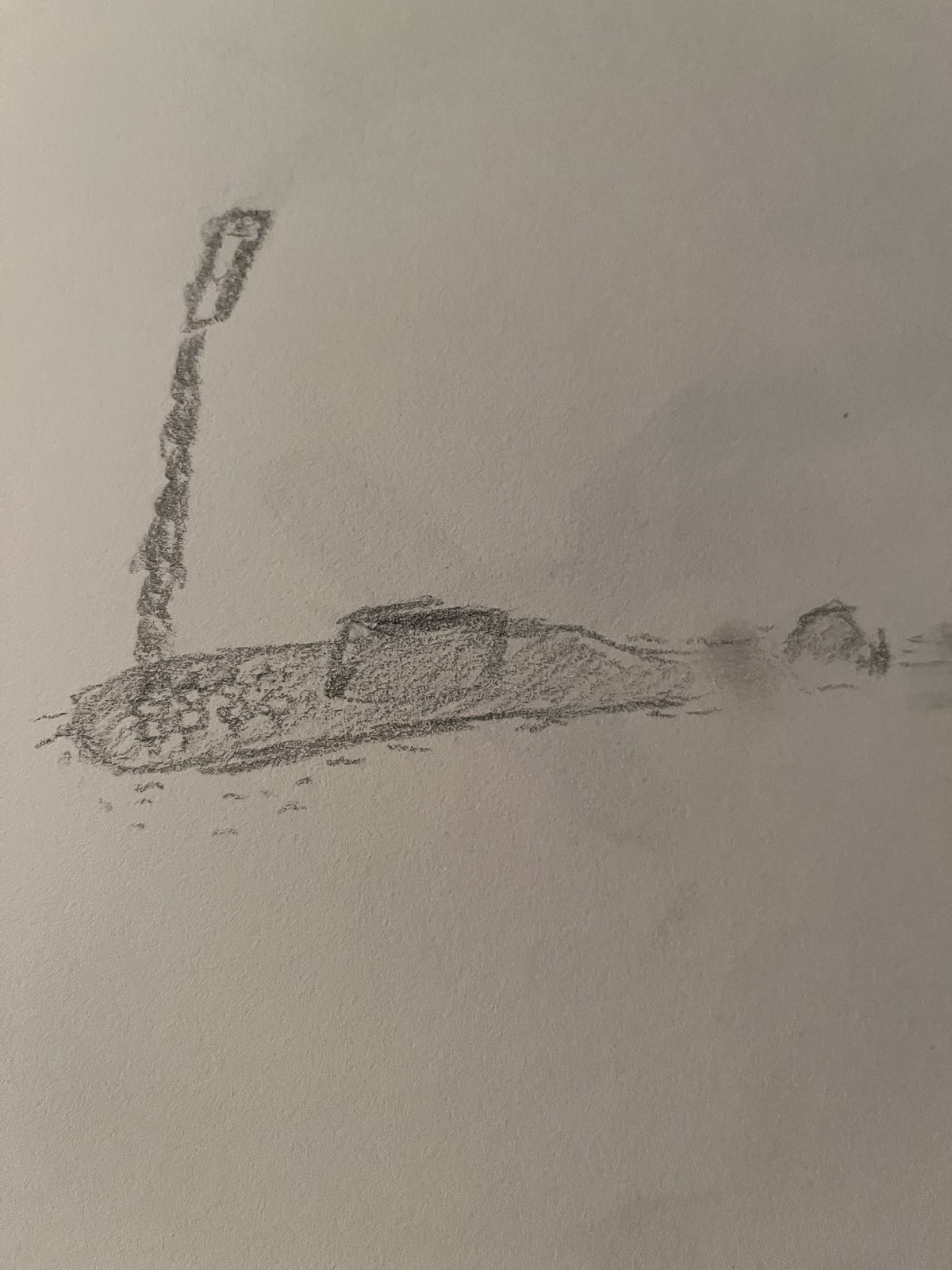This is a black-and-white, hand-drawn sketch on a gray piece of paper, depicted in a vertical, portrait-oriented image. The drawing is somewhat abstract and made with pencil, graphite, or black chalk. The central figure in the image ambiguously resembles both a submarine and a whale. On the left-hand side of the sketch, there's a spout releasing water, akin to a whale's blowhole but also suggestive of a submarine launching a missile. To the right, there is an elevated structure that could be interpreted as either the observation tower of a submarine or the "neck" area of the whale. Additionally, the far-right portion of the drawing includes a tail-like feature, supporting the whale interpretation. Overall, this hurriedly crafted sketch creatively blurs the lines between depicting a humpback whale swimming and a submarine in action.